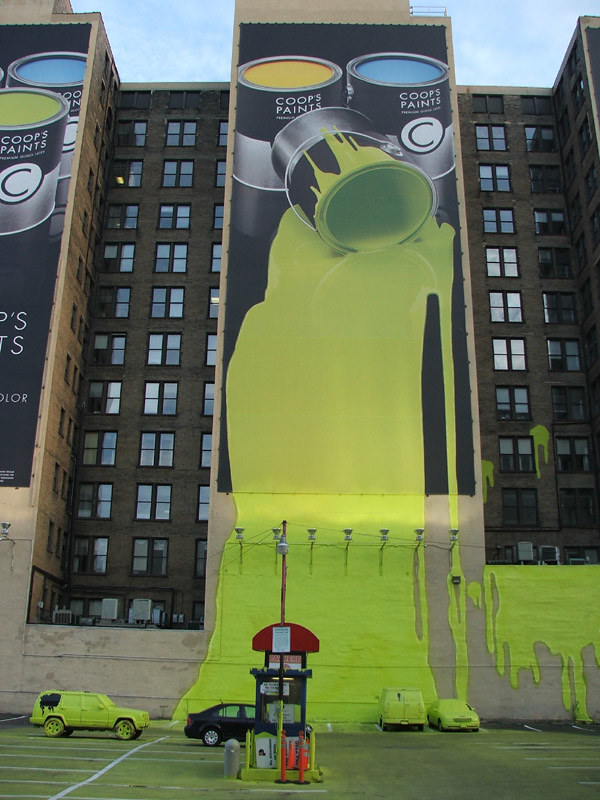This photograph, taken from within a large parking lot, captures a clever and visually striking Public Relations advertisement for Koops Paints. Dominating the scene is a high-rise building, approximately 10 to 12 stories tall, adorned with a massive mural featuring three humongous cans of paint in bright colors: yellow, blue, and green. The mural masterfully blends painted and real elements; the green paint can appears to have been tipped over, its contents spilling down the entire height of the building and extending onto the parking lot and several parked cars below. The spilled paint effect is so meticulously done that it seamlessly transitions from the large painted mural to real paint on the building and the vehicles in the lot, presenting an eye-catching and highly detailed visual spectacle. A ticket machine stands in the middle of the parking lot, adding to the realism of the scene.